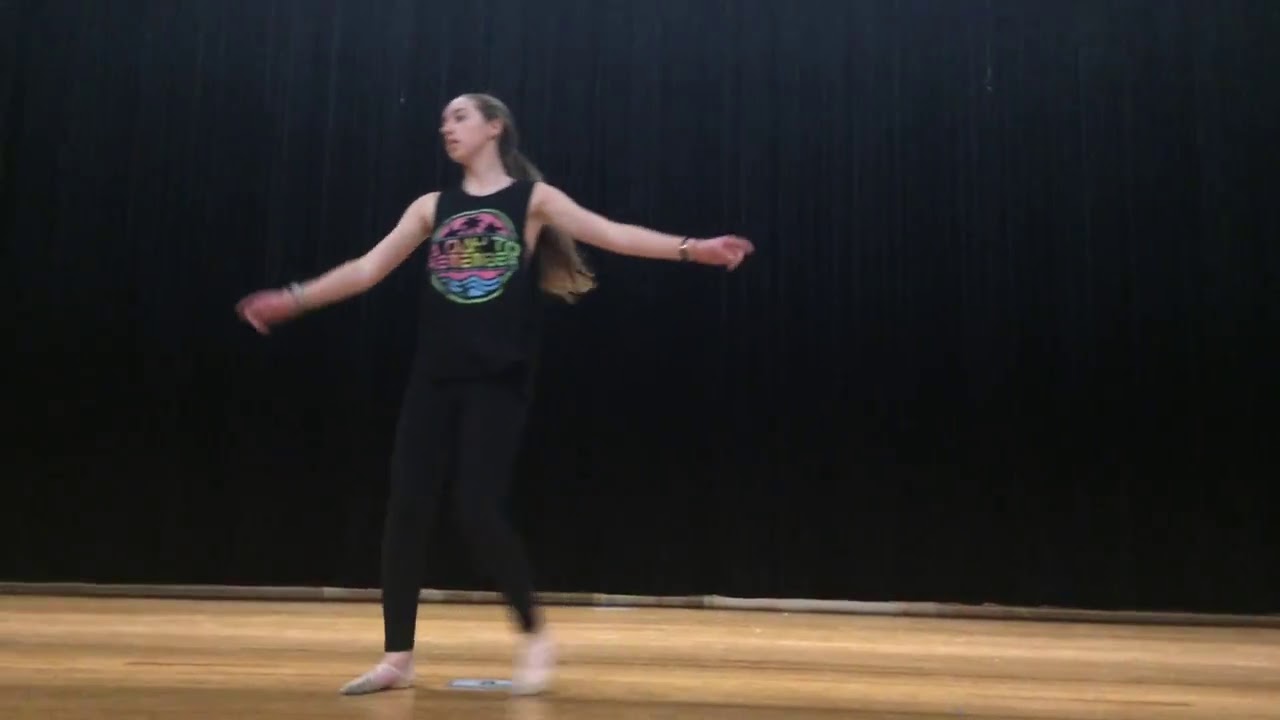The image captures a dynamic moment of a Caucasian girl in mid-dance, accentuated by slight motion blur. She stands slightly left of center on a high-gloss, golden wood floor, creating a striking contrast against the black curtain that forms the backdrop. The dancer is dressed in casual practice attire: a black tank top adorned with a circular, colorful logo in pink, blue, and green, paired with black leggings. Though the exact details on the shirt remain indistinct, the word "remember" is discernible. She wears form-fitting dance shoes, possibly ballet flats. Her arms are gracefully extended to her sides, while her dark brown hair, tied back in a ponytail, swings behind her. Visible accessories include a watch on her right wrist and a bracelet on her left. The girl's gaze is directed towards the left side of the image, suggesting she is about to pivot or twirl, captured in the fluidity of movement by the photographer.